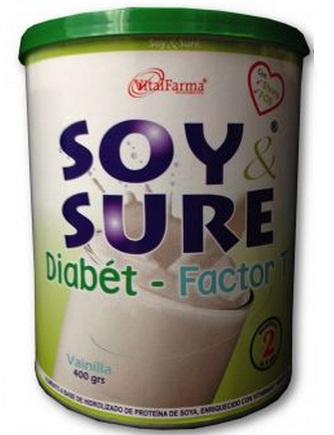The image displays a cylindrical product container with a green plastic lid. The top of the label features a thin green line, transitioning to white, and ending with a lime green color at the bottom. Prominently printed in red at the top is "Vita Pharma," alongside a heart symbol. "Soy Sure" is written in blue across the midsection. Below that, "Diabete Factor" is found in both green and blue text. A depiction of a white, milk-like substance splashing out of a glass further adorns the label, with "Vainilla," meaning "vanilla," noted underneath. The bottom left corner indicates the container holds "400 grs." The use of varied colors like red, blue, green, and accents like the heart symbol add to the detailed, vibrant design.